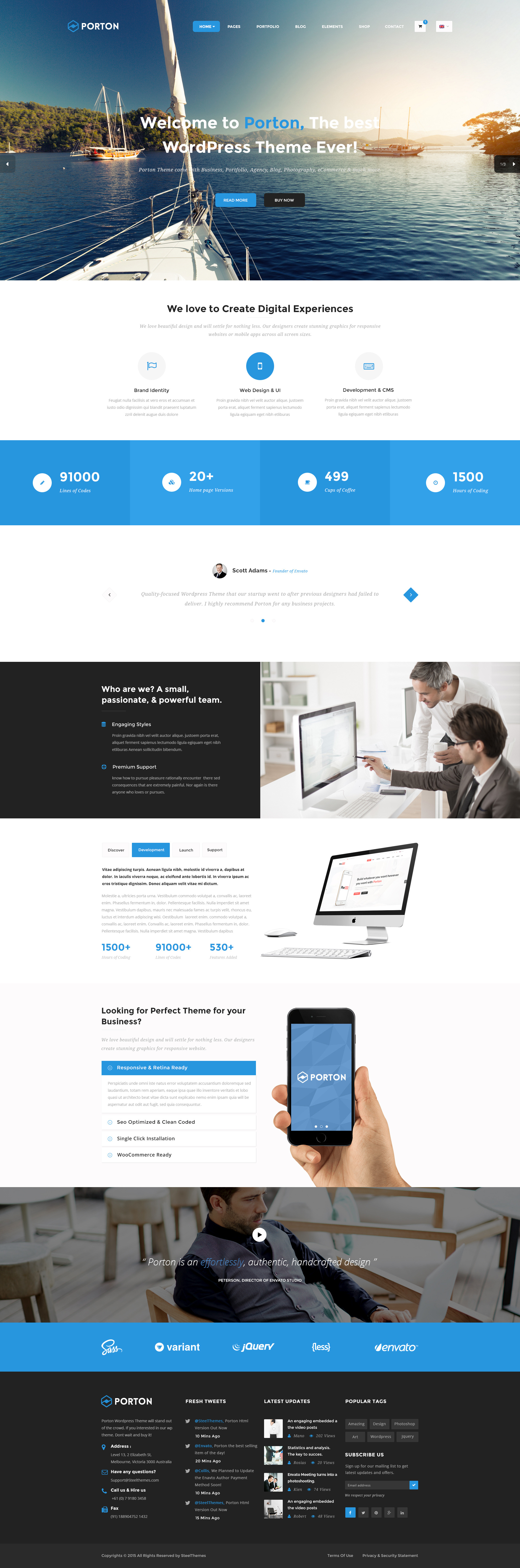This image captures the opening page of a website, albeit with some distortion when zoomed. Dominating the top section is a striking photograph taken from a sailboat, evidenced by the visible mast at the bow and surrounding safety lines. The calm waters stretch ahead, where a couple of other sailboats, identifiable by their masts, appear to be heading from a harbor into a larger expanse of water. The left side of the frame reveals a hint of land, while the right side showcases a solitary tree and, in the distance, a breathtaking sunset. Below the photograph, the text "We love to create digital experiences" is prominently displayed. Further down, various sections provide information about the site, featuring images of monitors, tablets, and other digital devices.